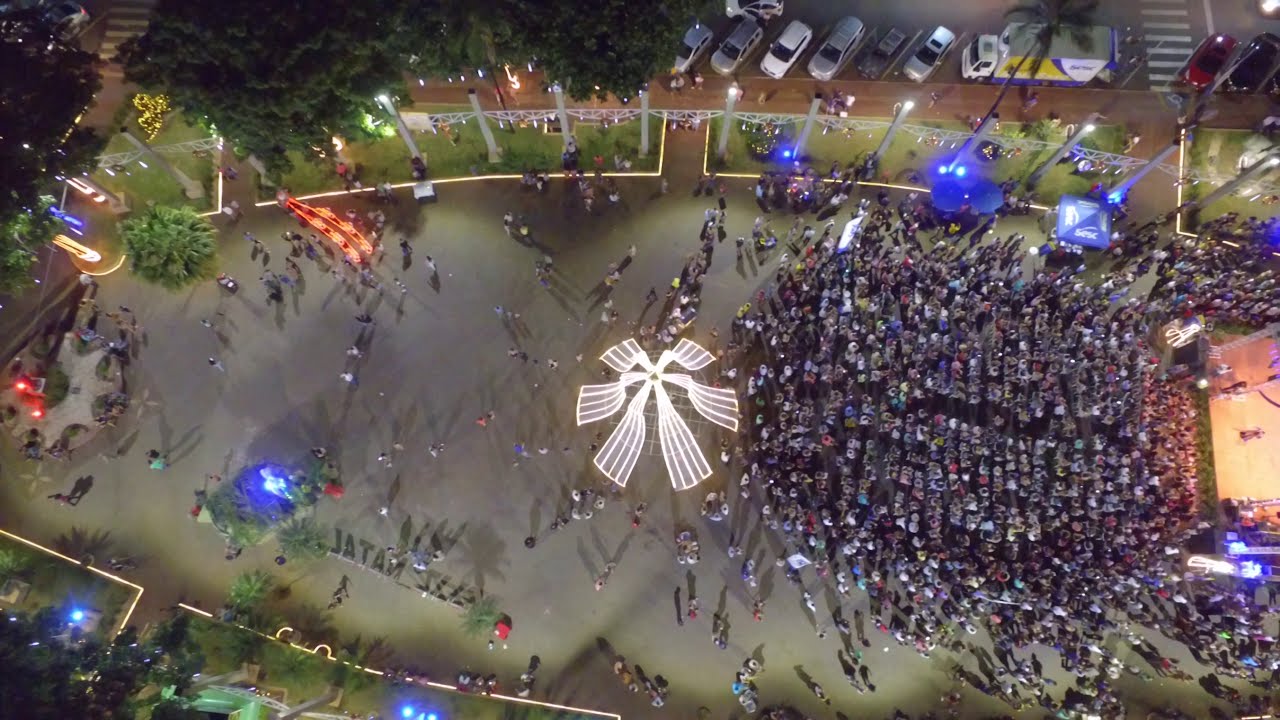The aerial photograph captures an evening concert at what appears to be a civic square or similar public space. The scene is dominated by a large, fenced-in concrete area, bathed in various lights, including blue, white, and yellow. The right side of the image shows a dense crowd, either standing or seated in rows, facing towards a stage which is partially visible. The stage area, outlined with brown metal railings and illuminated by blue and white lights, suggests a performance taking place. Central to the gathering is a large, white object resembling a fan, clearly visible in the midst of the crowd. Surrounding the main area, an illuminated white strip walkway frames the scene, with pathways leading in and out. Just beyond the fenced area, the upper right corner reveals a parking lot filled with cars and bordered by trees. The overall impression is that of a bustling event attended by numerous people, captured from a high vantage point.